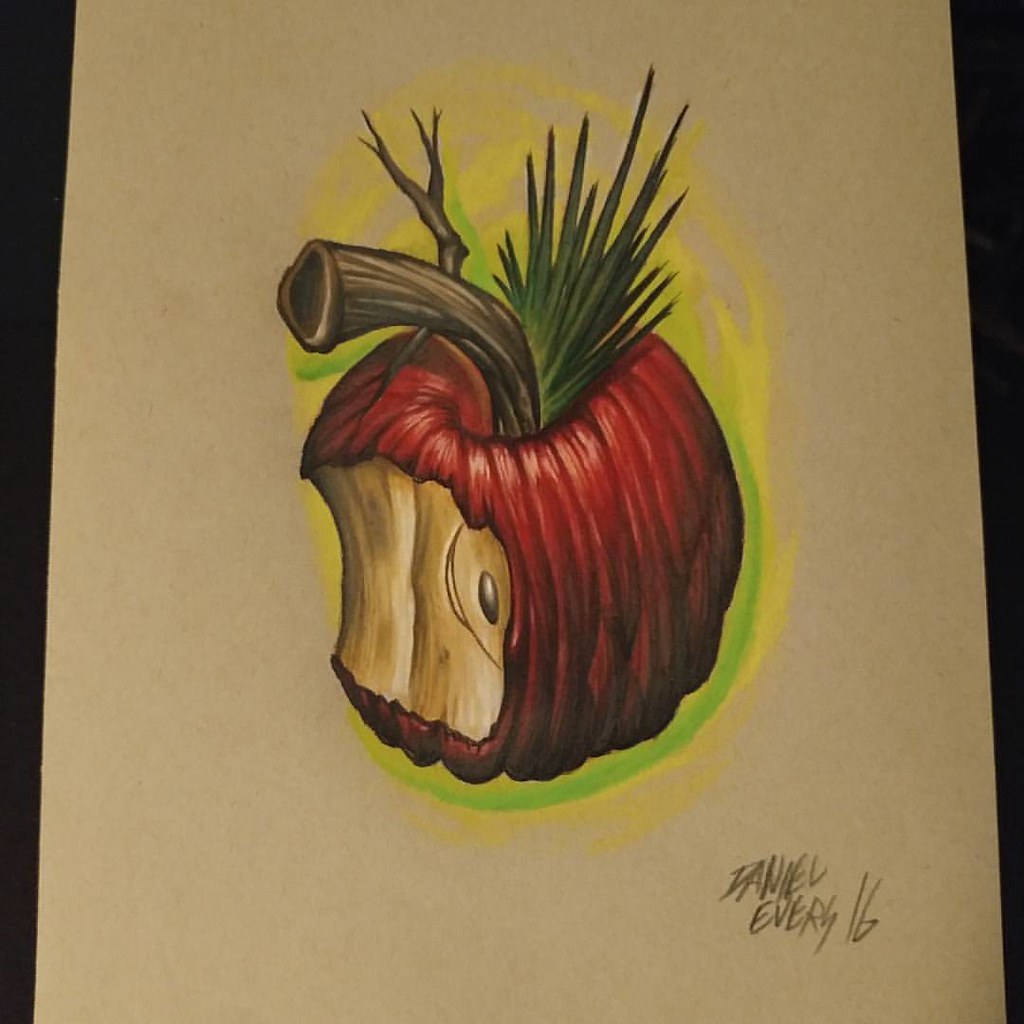This artistic drawing is rendered on a tan, almost brown, sheet of paper or canvas. The left and right edges of the image feature black stripes, likely indicating the tabletop or surface beneath the sheet. At the bottom of the image, a pencil signature reads "Daniel Every 16." 

The focal point of the artwork is a uniquely depicted apple. It features a bite taken out of it, revealing flesh that transitions from white to a browned hue. The apple's outer skin is a deep red with darker, almost black, accents at the bottom, giving it a distressed, striped appearance. A remarkably realistic wooden stem protrudes from the top, accompanied by small tufts of green grass.

Surrounding the apple is an ethereal, glowing effect in green and yellow hues that resembles flames, adding a surreal element to the composition. The combination of realism and abstract elements creates a visually captivating and thought-provoking piece.